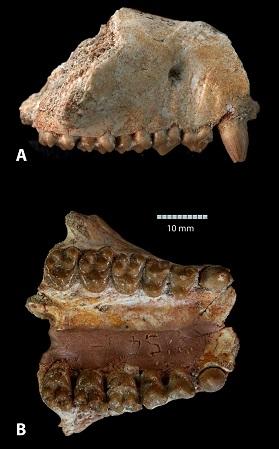The image displays two ancient artifacts labeled "A" and "B" against a black background, each representing fossilized remains of teeth and bones from what appears to be an animal. At the top, artifact "A" is a fragment that resembles a jawbone with a row of six old, dark brown teeth, distinguishable despite its rock-like appearance. The fragment in "A" shows significant wear and antiquity. Below it, artifact "B" is a more complete specimen, showcasing both the upper and lower sets of teeth, each with six teeth, suggesting a clearer representation of a mouth, though it also shows signs of great age and wear. A scale marker in the middle of the image reads "10 mm," providing context for the size of these artifacts, which are relatively small but intricate, with the largest tooth highlighted on the far right of artifact "B". The fossils' rough and jagged edges, particularly in "B", further emphasize their ancient and fossilized nature.